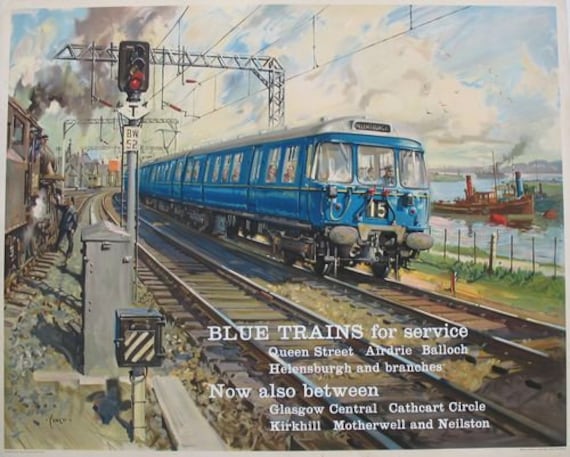The image is a vintage, landscape-format advertisement for a train service, done in an impressionistic or watercolor style. The illustration depicts a blue passenger train with the number 15 on the front, moving towards the right. To the right of the train is a body of water with a tugboat, and in the distance, several other boats are visible. On the left side, there's an empty train track curving into the distance alongside a brown train, with a man in a gray suit standing next to it. A signal light on a pole, displaying a red light with the letter T underneath, is seen nearby. Above the train, metal scaffolding stretches across the sky, which is blue with large white clouds. The white text at the bottom of the poster reads: "Blue Trains for Service, Queen Street, Airdrie, Bullock, Helensburg, and Branches. Now also between Glasgow Central, Cathcart Circle, Kirkhill, Motherwell, and Neilston."